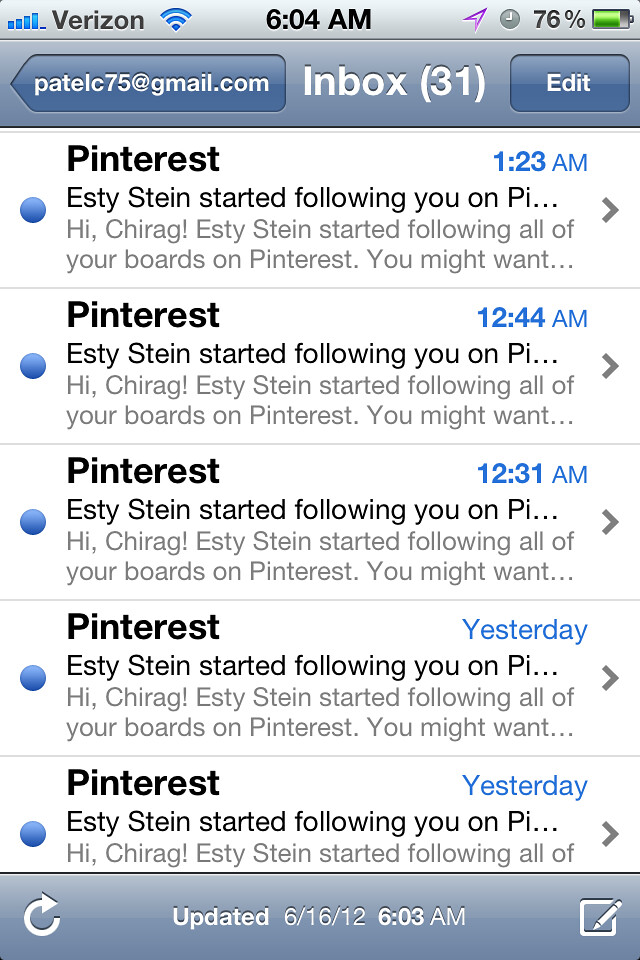The image is a smartphone screen capture of an Apple iPhone displaying a social media feed within a mail application. The very top section of the screen displays the phone's user interface, indicating a Verizon signal with four blue bars, a Doppler radar image, the time 6:04 AM, and a battery level of 76%. The email account shown is patelc75@gmail.com with an inbox count of 31 unread messages. The mail app interface includes a series of five unread emails, all originating from Pinterest, indicating that "Etsy Stein started following you on Pinterest," with timestamps ranging from 1:23 AM, 12:44 AM, 12:31 AM, and two labeled as 'yesterday.' The bottom of the image includes the standard mail app icons - a refresh icon on the bottom left, a timestamp indicating the last update at 6:03 AM on June 6th, 2012, in the center, and a compose email icon on the bottom right. The overall impression is a repetitive notification feed from Pinterest regarding a new follower named Etsy Stein.